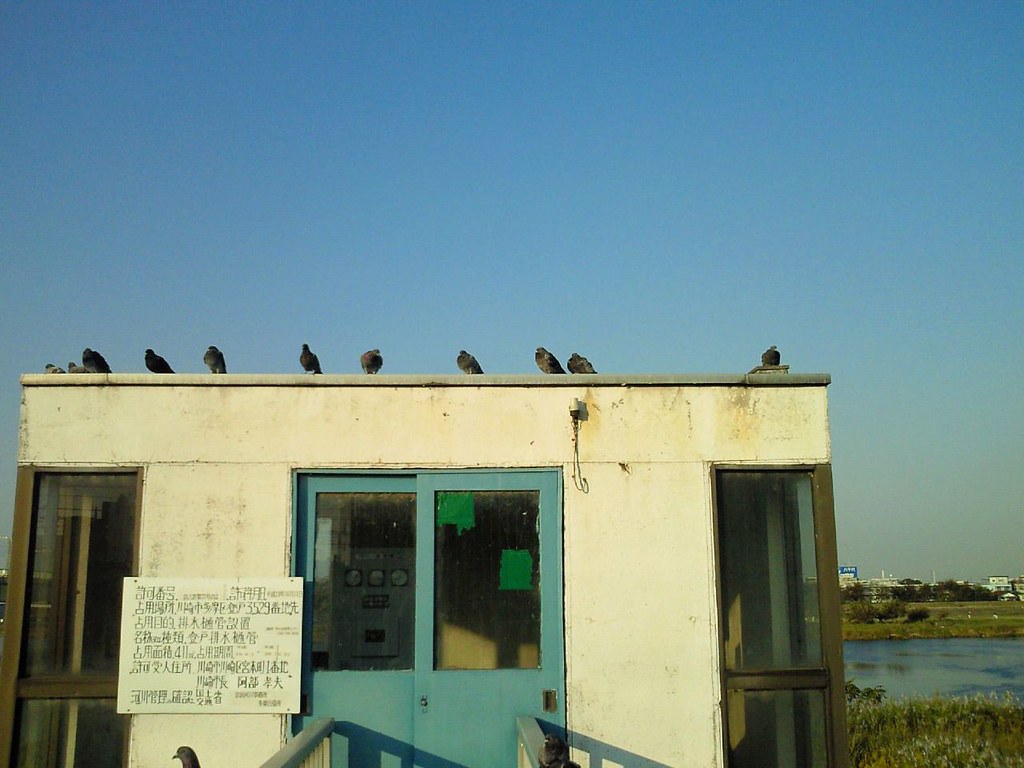The photograph captures a tranquil outdoor scene on a sunny day with a clear blue sky. At the forefront, there is an old, small, one-story building, noticeable for its stained white exterior and striking blue double doors. Each corner of the building features glass windows, and perched on the flat roof are approximately ten small, black birds, seemingly at rest. To the left of the door, a white sign with Asian characters hints that the photo may have been taken overseas. Surrounding the structure is a mix of green grass and marsh-like plants. Behind the building, a body of water, possibly a river or pond, adds to the serene landscape. In the far distance, a cluster of white buildings is visible on the horizon, completing this picturesque setting.